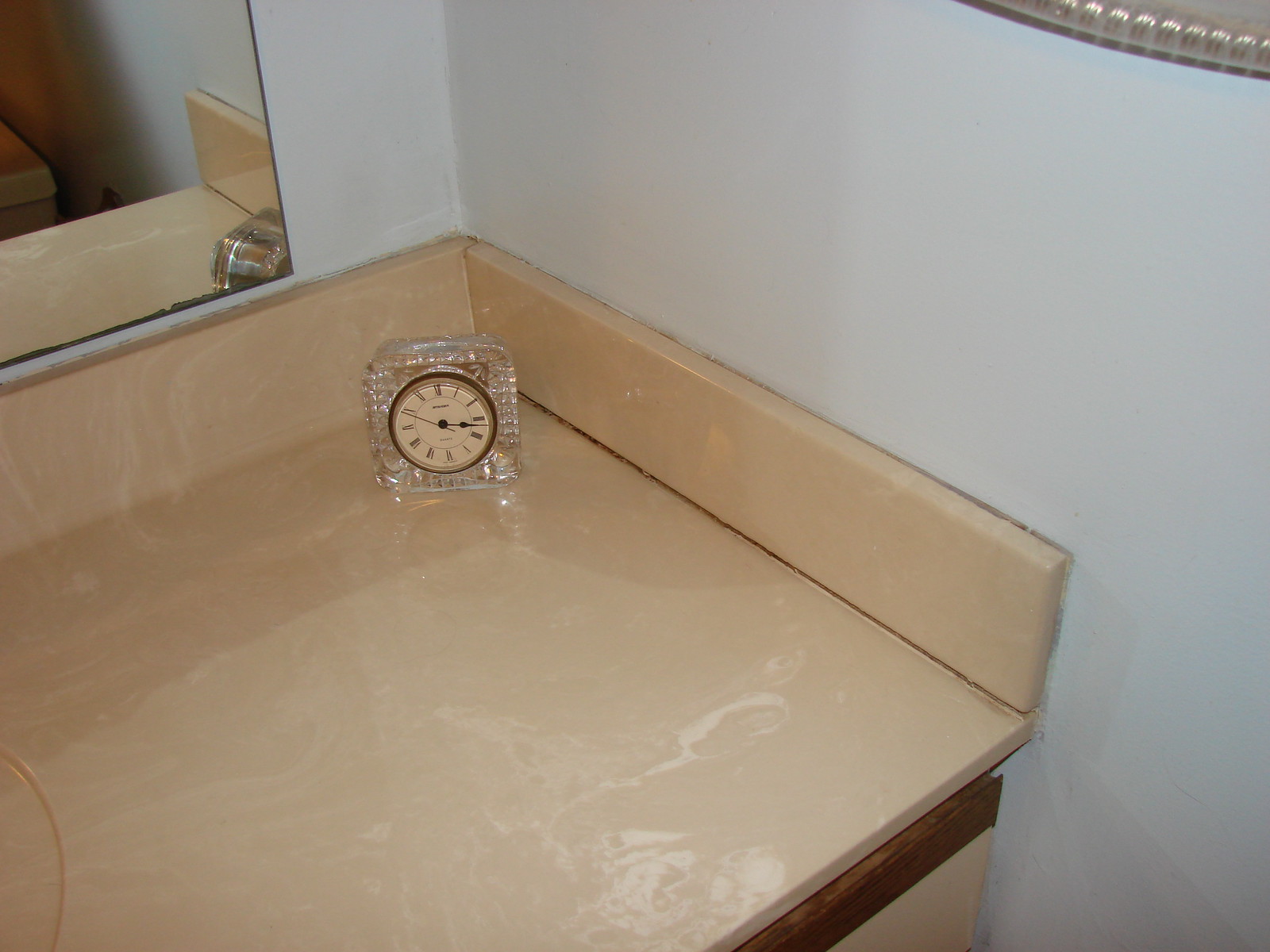A detailed close-up of a bathroom counter showcases a sophisticated tan marble surface with coordinated trim. In the upper corner of the counter, a clock is elegantly positioned. The clock features a face in a harmonious tan shade that matches the marble, complemented by a sleek brown rim, adding a touch of classic charm to the tasteful bathroom decor.